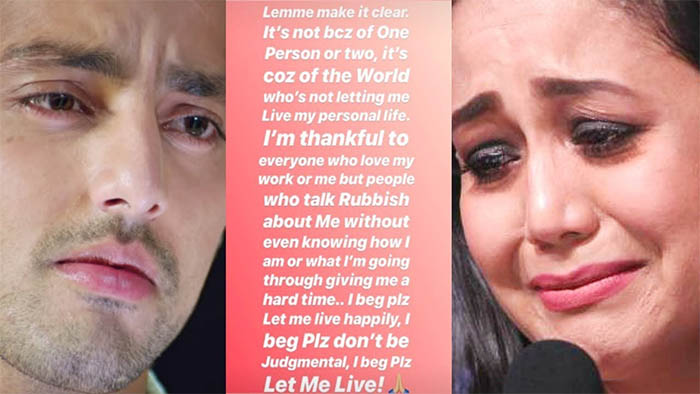The image is divided into three sections: on the left is a close-up of a sad-looking Caucasian man with a five o'clock shadow, facing roughly the 5:30 position. On the right, a Caucasian woman with long dark hair, makeup, red lipstick, and a microphone in front of her mouth is facing roughly the 6:30 position, also appearing sad. Both close-ups capture their facial expressions from their chins to the middle of their foreheads. Between them, there is a pinkish-peach background with white text running vertically. The text reads: "Let me make it clear, it's not because of one person or two, it's because of the world who's not letting me live my personal life. I'm thankful to everyone who loves my work or me, but people who talk rubbish about me without even knowing how I am or what I'm going through are giving me a hard time. I beg, please let me live happily. I beg, please don't be judgmental. I beg, please let me live."

This image effectively conveys a plea for understanding and a call against judgment, reflected in the somber expressions of both individuals and the earnest text in the center.